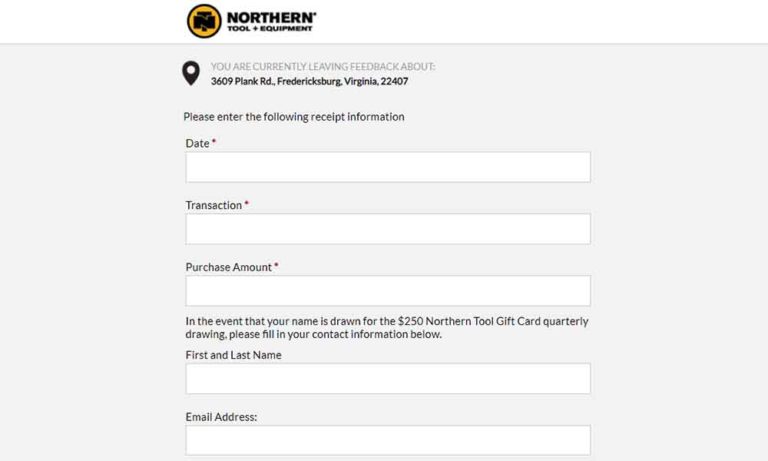Image Description:
The image displays a feedback webpage from Northern Tool and Equipment, specifically for a location at 3609 Plank Road, Fredericksburg, Virginia, 22407. The website is designed for customers to leave feedback regarding their experiences. It requests various pieces of information, including the date, transaction details, purchase amount, and contact information for entry into a quarterly drawing for a $250 Northern Tool gift card.

The background of the webpage is a clean, eggshell white, contributing to a minimalist and uncluttered appearance. Most of the text is black, ensuring readability, with the exception of the phrase "you are currently leaving feedback about," which appears in a subtle light gray. Highlighting the branding, the Northern Tool and Equipment logo stands out in an orange-yellow, macaroni-like color. The logo features a black circle with an 'NT' insignia at its center.

The text input fields for entering feedback and personal details are plain white, maintaining the page's simple aesthetic. Required fields are marked with small red asterisks. Overall, the page conveys a straightforward layout typical of customer feedback forms, focusing on functionality and ease of use. The image does not include options for editing details, which might be accessible either further down the page or on a subsequent screen.